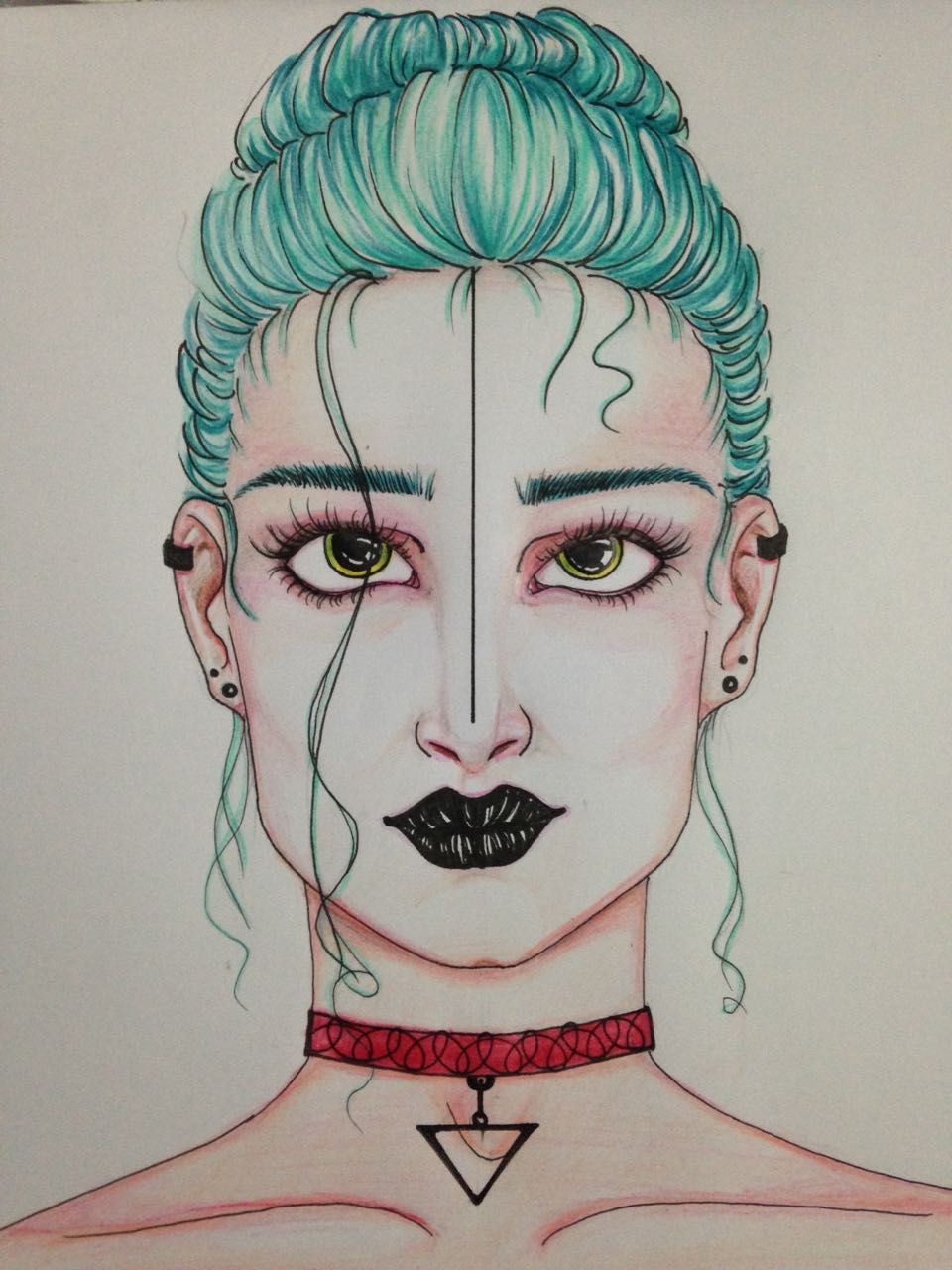This detailed artistic drawing features a captivating portrait of a woman facing the viewer. Her gaze is directed upwards, revealing striking yellow, gold-like eyes that exude a sense of mystique. She sports a unique hairstyle, with teal-colored hair elegantly styled into a bun. Wisps of hair can be seen trailing down the back of her head and framing her face.

Her lips are adorned with bold black lipstick, emphasizing her enigmatic expression. Around her neck, she wears a distinct choker that is vivid red, adorned with a hanging black, upside-down triangle pendant, adding to her avant-garde appearance.

The artwork is richly colored, and her skin is rendered in a delicate light rose hue, with subtle shading enhancing the contours of her face and body. Her ears are adorned with multiple piercings: the tops bear small black clip piercings, while her earlobes each feature two circlet piercings, one set on each side. This intricate and colorful portrait combines bold and delicate elements, creating a compelling and richly textured image.